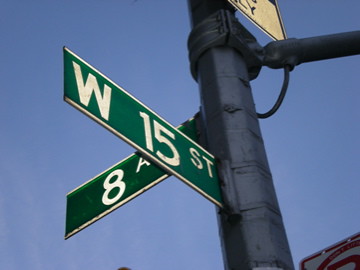The image depicts a thick utility pole with two intersecting street signs photographed from a low angle, giving the view an upward perspective. The prominently visible street sign extends outward at an angle and features a dark green background with white borders at the top and bottom, displaying "W 15 Street" in bold white text. Behind this sign, there is a perpendicular green street sign, partially visible, marked with a white-bordered "8" and a small letter "a." Additional fixtures on the pole extend out of the frame, including the bottom edge of a white sign. The backdrop is a clear blue sky, indicating a bright, cloudless daytime. In the bottom right corner of the image, a sliver of another street sign is attached to the pole, showing hints of red and white, though its details are not fully visible.